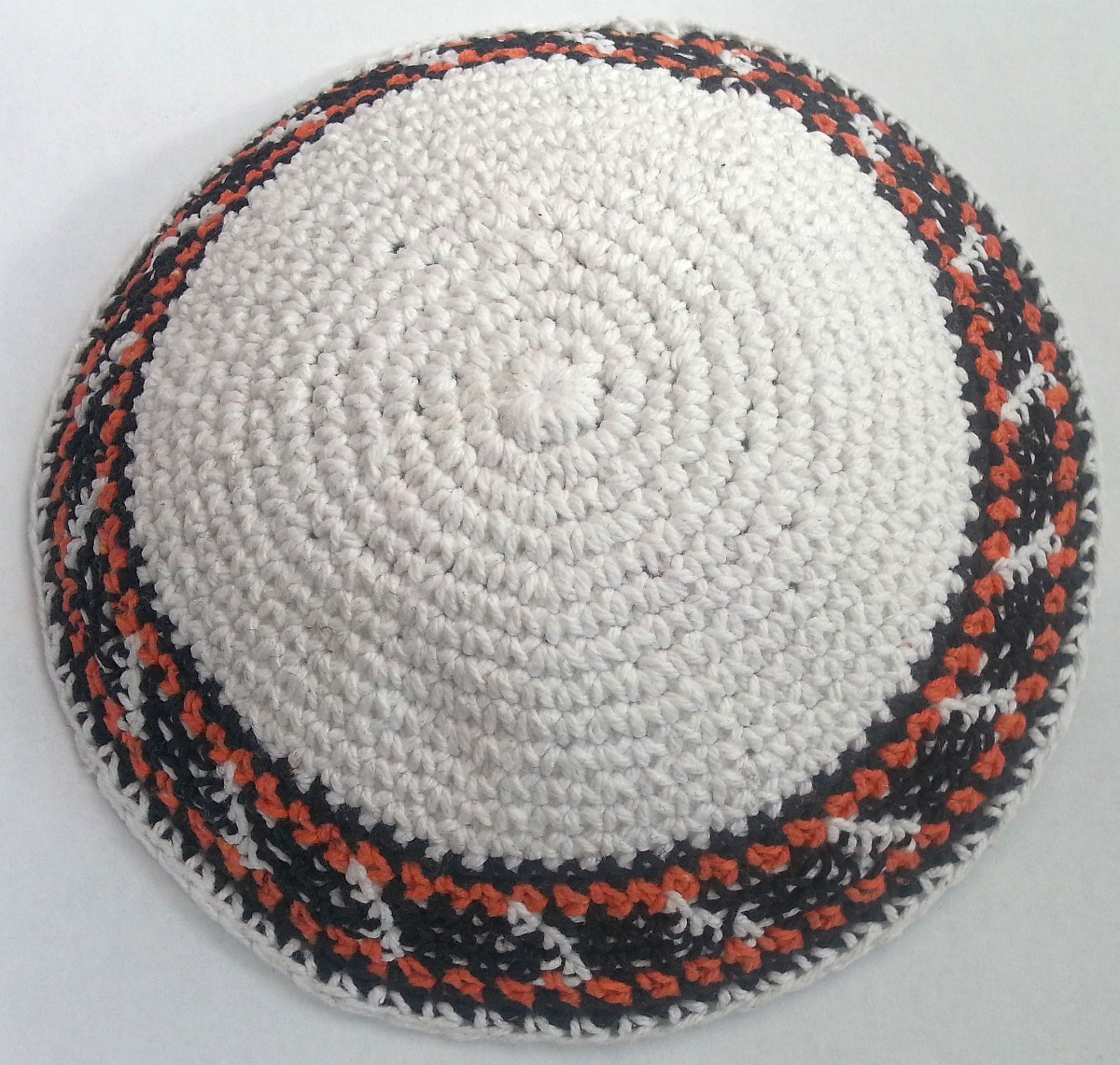The image captures a detailed, handmade circular knitted or stitched material set against a solid light gray background, occupying most of the frame. Predominantly light beige in color, the centerpiece of the item is a pure white circle. Encircling this white center, the design features alternating rows of black and orange layers, creating a distinct spiral pattern that radiates outward. The intricate craftsmanship of this piece suggests it might be a decorative placemat or the base of a basket, with the seamless, repeating color pattern highlighting the meticulous and deliberate stitching. There is no text or writing present in the image.